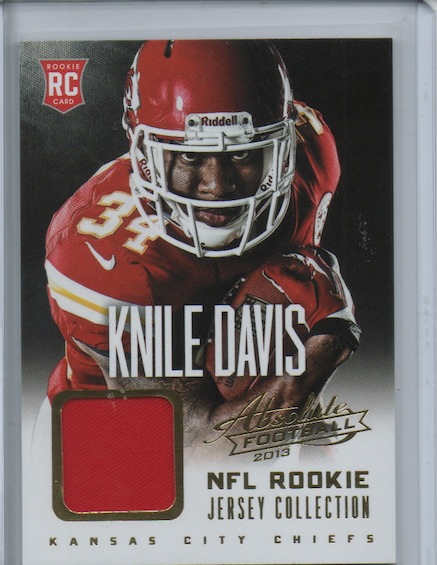This trading card from the 2013 NFL Rookie Jersey Collection features Nile Davis of the Kansas City Chiefs. The card's design includes a gray border and prominently displays Davis in his red Chiefs uniform, complete with a red helmet featuring the KC Arrowhead logo and a white face guard. He wears the number 34 in white with a yellow outline, signaling his position as a running back. The knee-length shot captures Davis holding a football, poised as if ready to run. At the center of his torso, his name "Nile Davis" is printed in white. The card is marked with various inscriptions, including "Absolute Football 2013" and "Rookie Card," with the lower right corner specifically indicating "Absolute Football 2013 NFL Rookie Jersey Collection" and "Kansas City Chiefs."